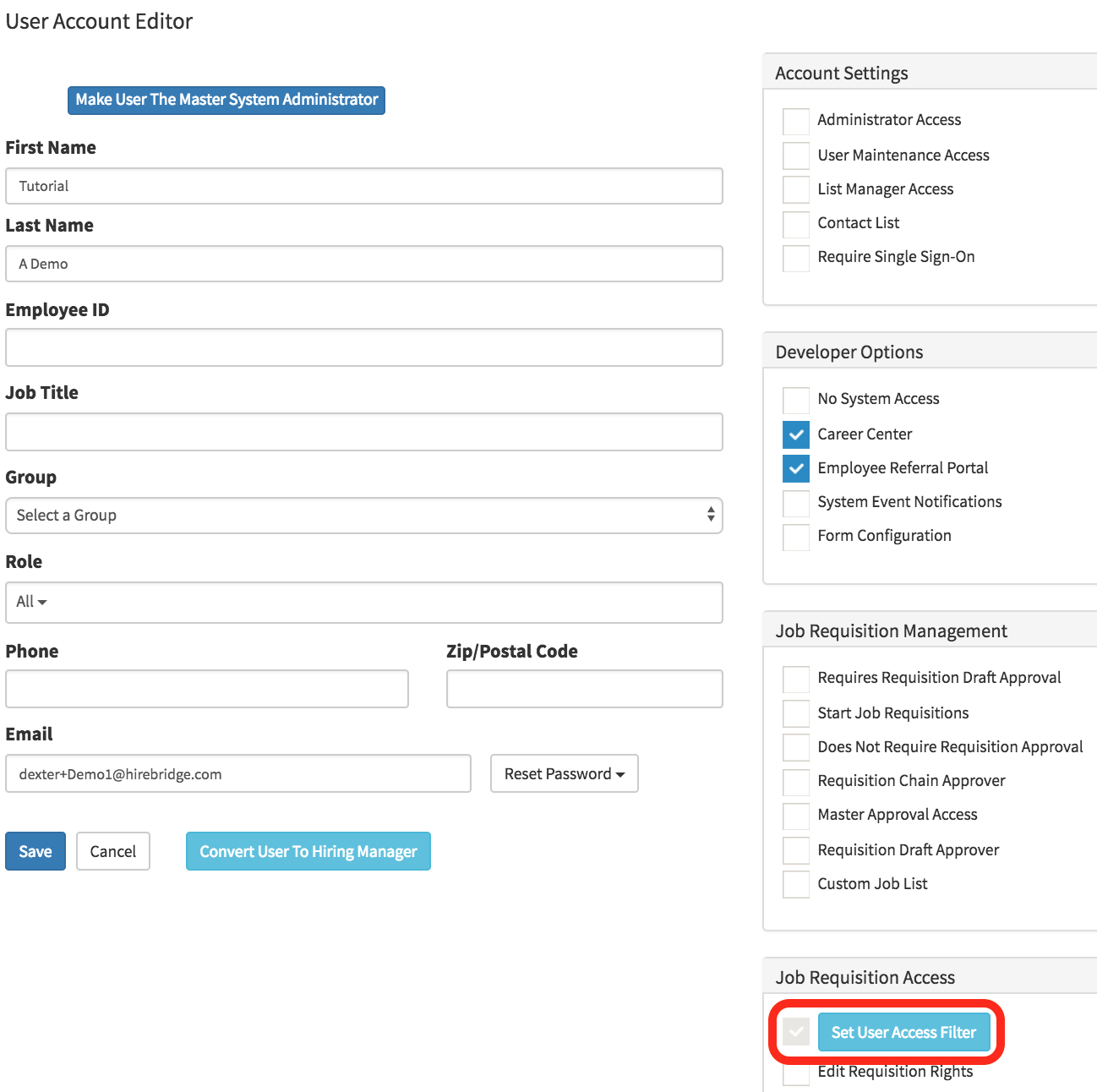This image depicts a user profile within an account editor interface for a specific app or website. The screenshot provides a detailed view of the fields and options available for editing the user account. 

At the top of the form, users can modify various pieces of personal information such as the "First Name," which is filled in as "Tutorial," and the "Last Name," filled in as "Demo." Additional fields include "Employee ID," "Job Title," "Group," which features a dropdown selection indicated by an upside-down triangle, "Role," another dropdown selection, "Phone," "Zip/Postal Code," and "Email." The email field in this example is filled out as "dexter.demo1@hirebridge.com."

Below the email field, there are options to manage the account's password and save or cancel any edits. The "Save" button is blue, while the "Cancel" button is white. Users also have the option to convert the user to a "Hiring Manager," which is displayed as a light blue button.

Prominently displayed is a rectangular blue button with white text labeled "Make User the Master System Administrator," suggesting an action to elevate user privileges. 

To the right of the main form, there's a side column with multiple categories for further account customization, including "Account Settings," "Developer Options," and "Job Requisition Management." Each category contains additional sub-options.

At the bottom of the sidebar, there's a highlighted option in red labeled "Set User Access Filter," likely indicating an important or urgent setting related to the user's access permissions. This detailed layout offers comprehensive tools for managing and editing user information and permissions within the system.